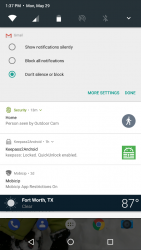The image appears to be a screenshot from a smartphone. Here is a more detailed and cleaned-up caption:

---

The screenshot displays a smartphone interface at 1:31 p.m., indicated in the upper left corner. Adjacent to this timestamp are various status icons, including signals for Wi-Fi, cellular bars, battery level, and Bluetooth. The screen showcases a drop-down menu, with a prominent Gmail icon on the left side.

Below the Gmail icon are three circular buttons, each with associated text that is partially obscured. The options appear to relate to sharing notifications and blocking or managing certain features, with the bottom option highlighted in green. Towards the bottom right of this menu, there are two green buttons labeled "More Settings" and "Done."

Further down the screen, the image quality diminishes, making some text unreadable due to poor resolution and low contrast. However, it is clear that "Fort Worth, Texas" is written in white font over a black strip at the bottom of the screen, accompanied by a sun icon and a temperature reading of 87 degrees.

The navigation bar at the bottom of the phone shows several icons: a blue circle with a white phone for calls, a blue circle with a person icon for contacts, and a white circle with two rows of three dots each. There's also a colorful Google search button in red, yellow, green, and blue, along with a black circle on a blue background and a left-pointing arrow.

---

This caption attempts to convey all the elements seen in the screenshot clearly and comprehensively.